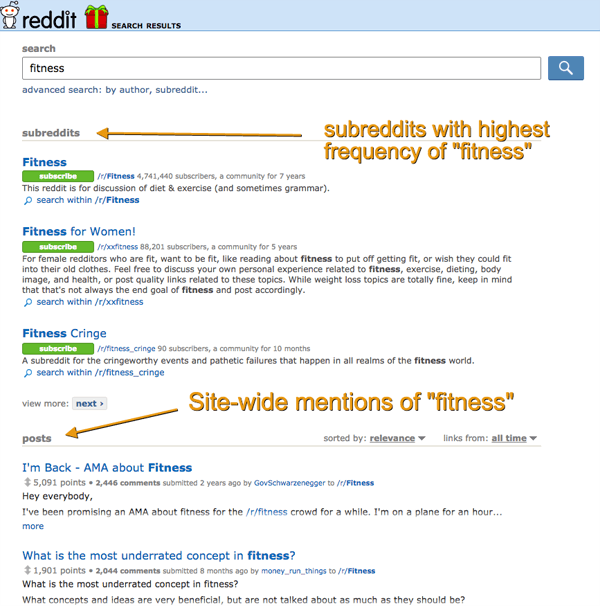This screenshot showcases the homepage of the Reddit website. At the very top, there is a light blue navigation bar. On the top left corner, the Reddit mascot is prominently displayed next to the word "reddit." Adjacent to this is a red icon with a green ribbon, followed by the heading "Search Results."

Directly below this header, a search bar section is evident. Above the search bar, the label "Search" can be seen, and within the search bar, the typed word "fitness" is visible. To the far right of the search bar, a blue box with a white magnifying glass icon represents the search function.

Below the search bar, the word "subreddits" is displayed, with a yellow arrow pointing from right to left accompanied by the yellow text "subreddits with the highest frequency of fitness."

The section below features bold titles, including "fitness," with descriptive text underneath. A prominent green "subscribe" button is also present.

At the bottom of the page, there is a callout labeled "sitewide mentions of fitness" with a yellow arrow pointing toward posts. Below this, two sections of text are visible, with the first line in bold blue text and smaller text underneath. These sections likely contain further details and context from Reddit posts.